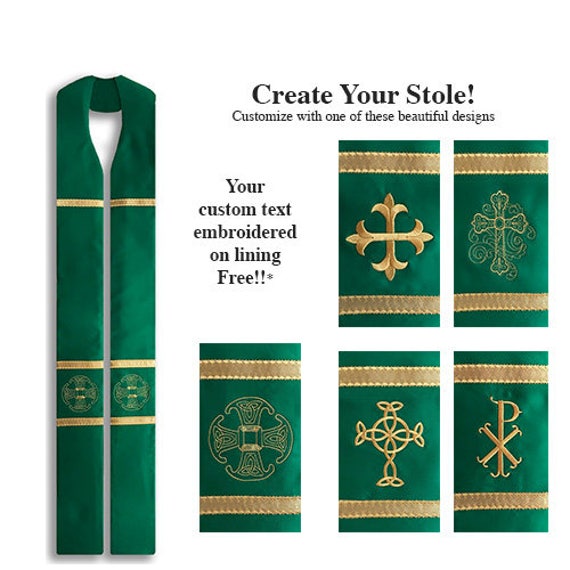This advertisement, displayed against a clean, white background, prominently features the bold, black caption "Create Your Stole" at the top, followed by the subheading "Customize with one of these beautiful designs." The advertisement showcases green velvet stoles, each adorned with gold stripes at the top and bottom. A detailed description alongside the stoles reads, "Your custom text embroidered on lining free!!*." 

To the left, there's a long, thin stole embellished with a gold stripe at the top, followed by two gray stripes, and a central Celtic cross design. Additionally, an image of five similar rectangular stoles is displayed, all echoing the green and gold theme and each featuring a unique Celtic cross embroidery in the center. This product appears to cater to religious apparel, possibly for clergy, and emphasizes customization and premium quality.